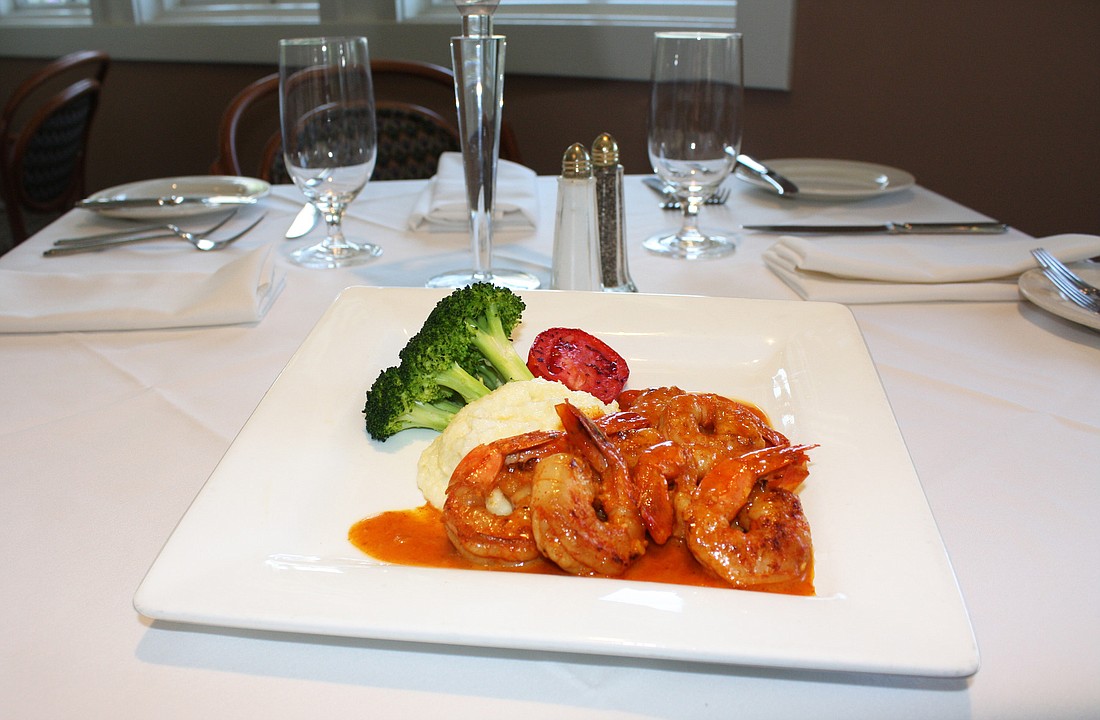The image captures a square dining table, likely in a restaurant, adorned with a crisp white tablecloth and matching white napkins. Dominating the foreground, there is a white square plate colorfully arrayed with a culinary ensemble: on the left side, a piece of steamed broccoli accompanies a small grilled tomato half, nestled next to a mound of mashed potatoes. Several pieces of shrimp, bathed in a reddish-orange sauce, are elegantly draped over the potatoes. Behind the plate, there are symmetrical place settings on either side, each equipped with two forks, a butter knife, a small plate, and a clear water glass. A salt and pepper shaker stands centrally, adding a touch of practicality to the scene. The backdrop features a brown wall accented with a brown chair with black woven material and the base of some white windows, providing a cozy yet refined atmosphere.